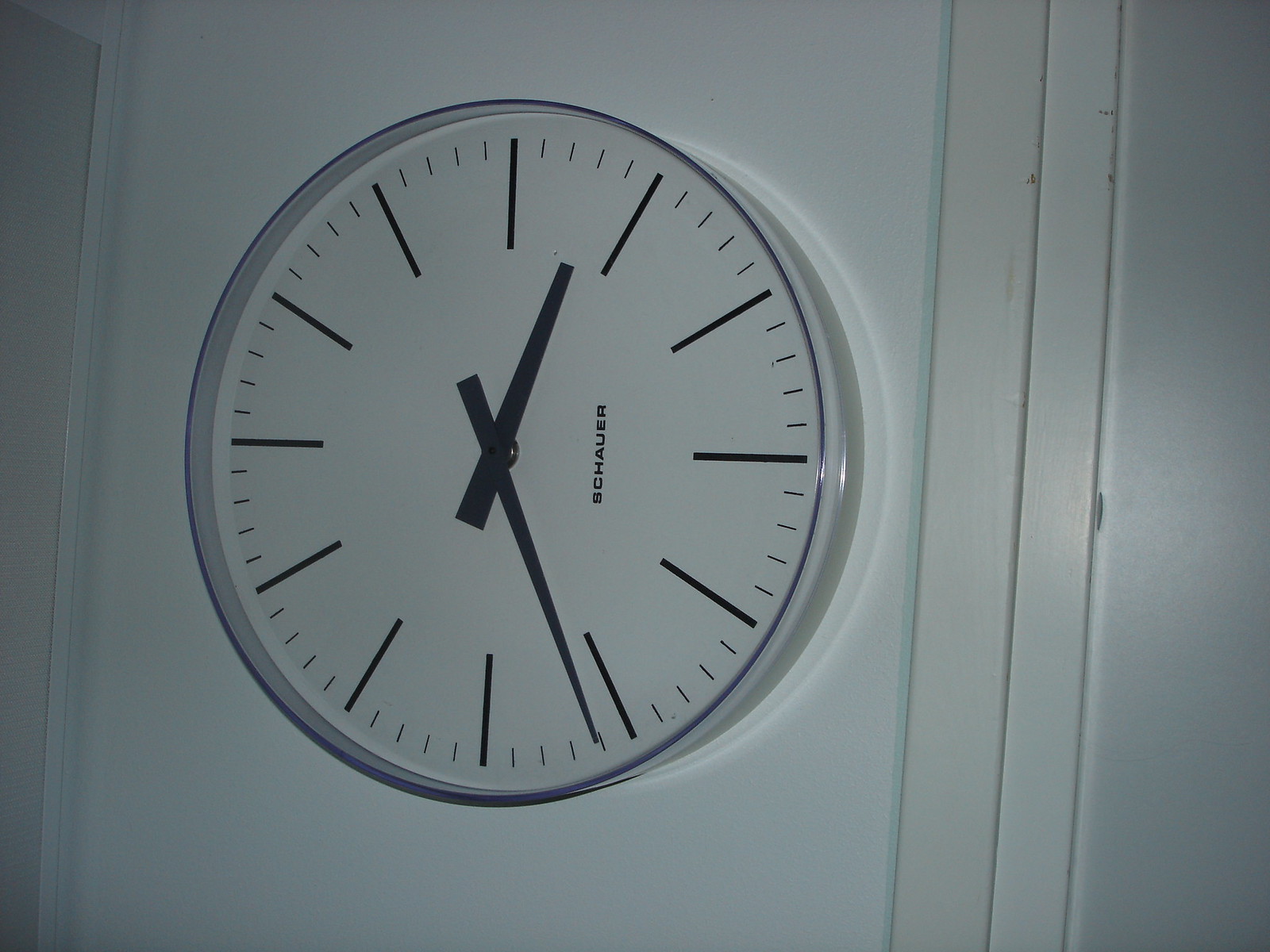This image depicts a sophisticated, modern clock mounted on a pristine white wall. The clock features a sleek, circular design framed by a thin metallic border. Its minimalist white face is distinctly marked with the brand name "ASHAUER" displayed vertically along the clock's center axis, suggesting that the clock might be photographed on its side. Instead of numerical markers, the clock face is adorned with twelve bold, evenly spaced rectangular bands indicating the hour positions. Interspersed between these are twelve smaller black bands demarcating the minutes. The hour hand is broad, tapering into an elongated trapezoidal shape, while the minute hand, svelte and pointed, offers a graceful contrast, harmonizing with the clock's overall elegant aesthetic.